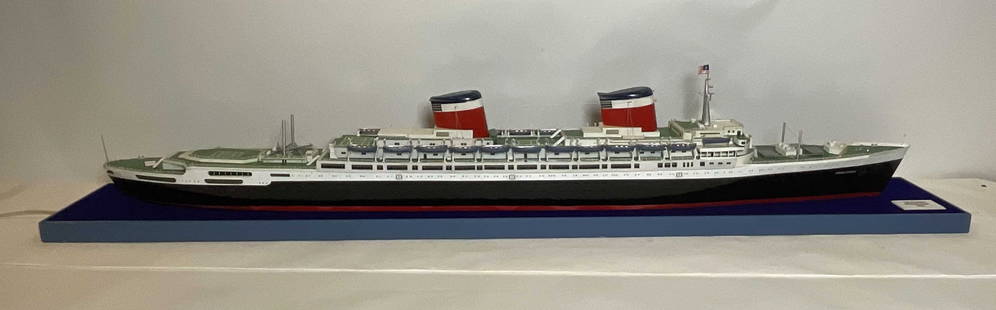This color photograph features a detailed model of a mid-1950s steamship, likely a passenger liner, displayed in a museum setting. The ship is mounted on a white and blue base, which rests on a white table against a light gray background. The steamship's elongated hull is predominantly black with a red keel and a white strip running along the top near the deck, which appears to be about two stories high. Prominently, the ship has two smokestacks designed in the traditional steamship style, with bases painted red, white stripes, and black tops, with the front stack slightly taller than the rear. Numerous windows are visible along the ship's white upper structure, and lifeboat rafts are positioned along the deck. At the front of the ship, a tall mast flies a flag, likely equipped with weather and communication instruments. The photograph captures the model in a realistic, representational style.